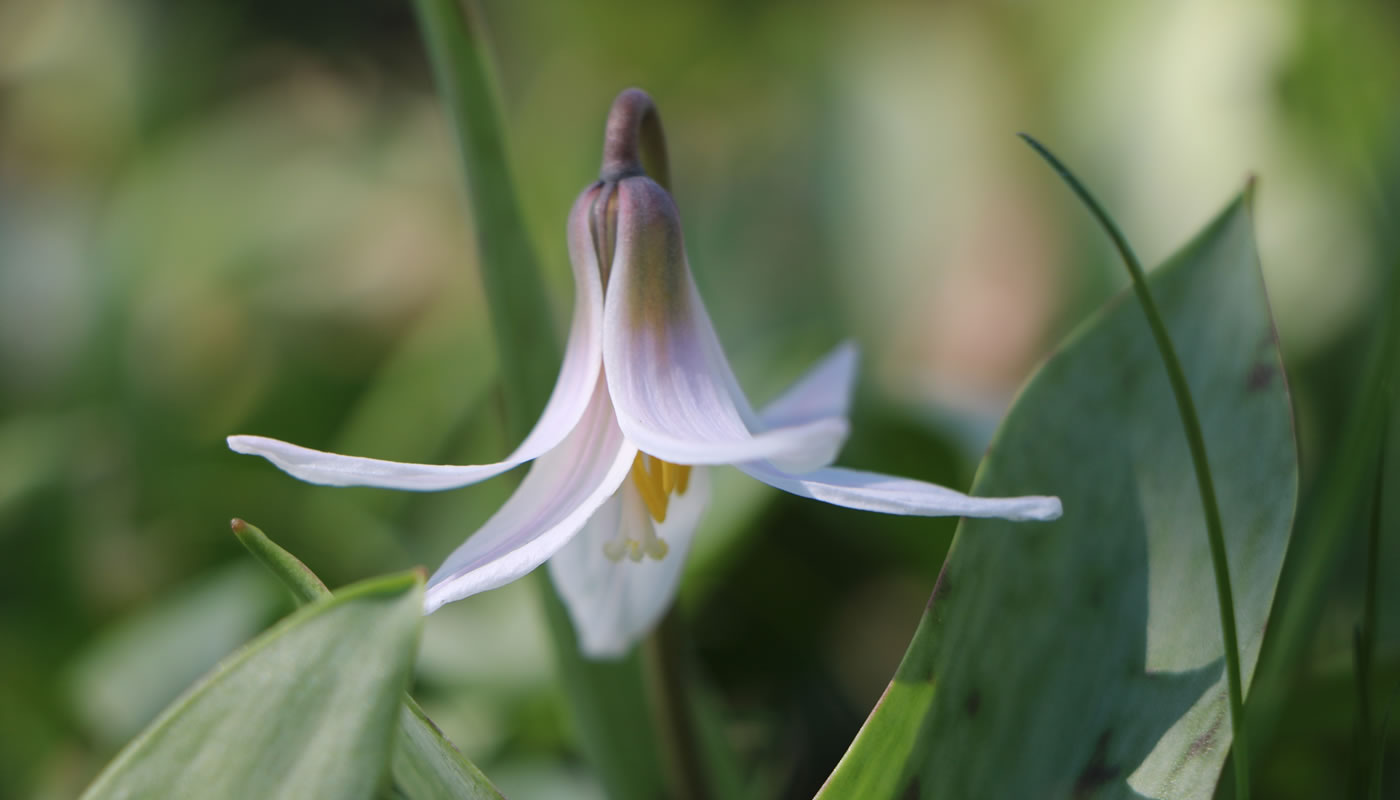The image features a delicate white flower hanging upside down with its stem bent in the shape of a cane, likely due to the flower's weight. The petals, predominantly white at the tips, gradually turn a soft purple as they approach the center. The flower's yellow, hair-like stamens droop downward, enhancing its unique allure. Flanking the flower, thick, dual-toned green leaves contrast beautifully with their dark and light greens, the one on the right cast in partial shadow with light filtering through its bottom. A slender green stem rises on the right before curving back to the left near the top. The out-of-focus background comprises green hues, with subtle hints of white and orange splotches, adding depth but not distracting from the central flower and leaves.